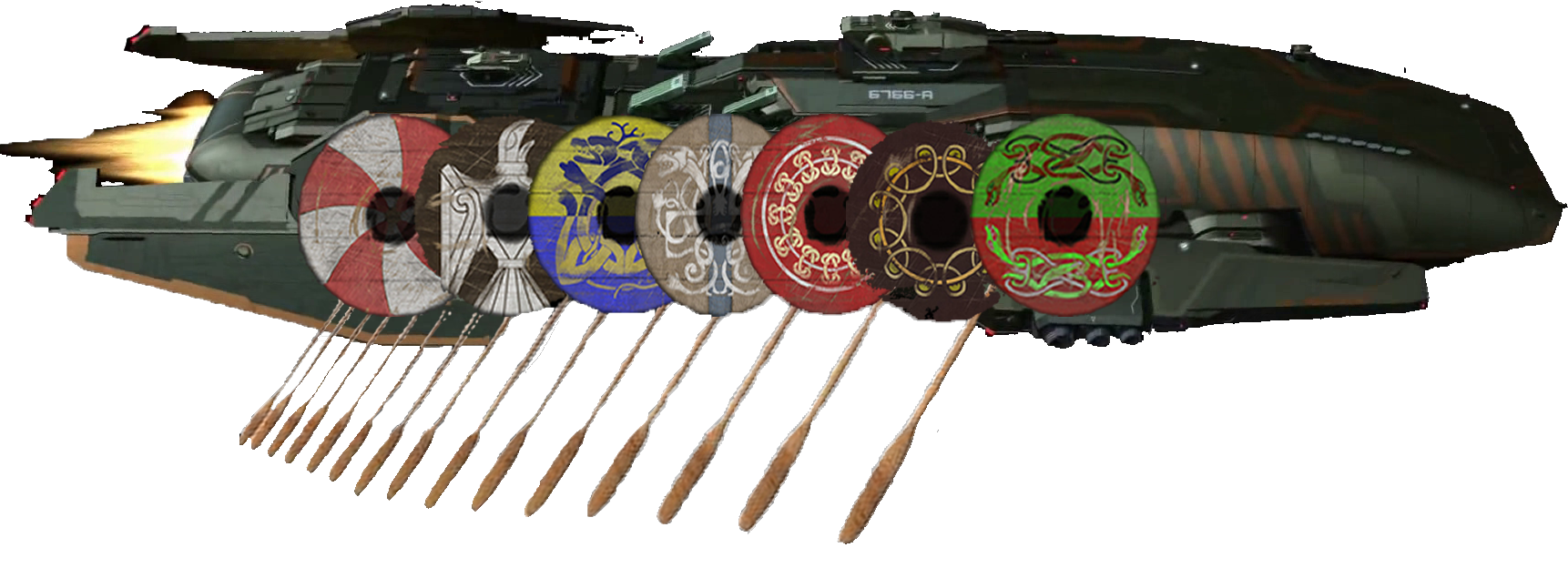This intricate artwork combines futuristic and historical elements in a captivating composite image. The centerpiece is a streamlined, dark green military spaceship with copper stripes adorning its front and sides. From the back engine, vibrant jet fire propels the craft forward. Along the sides of the spaceship, a series of round, wooden Viking shields are meticulously painted with various designs, including pinwheel patterns, intricate swirls, and stripes, in an array of colors such as white, red, black, yellow, and blue. Nestled among these shields are Viking motifs, including a detailed eagle and knot patterns, enhancing the historical influence. From behind the shields, wooden oars jut out, providing a stark contrast to the advanced, sealed hull of the ship. Atop the vessel, there appears to be a mounted gun, further emphasizing the blend of modern military technology with ancient Viking aesthetics. This artwork masterfully merges the past and future, creating a visually compelling narrative.